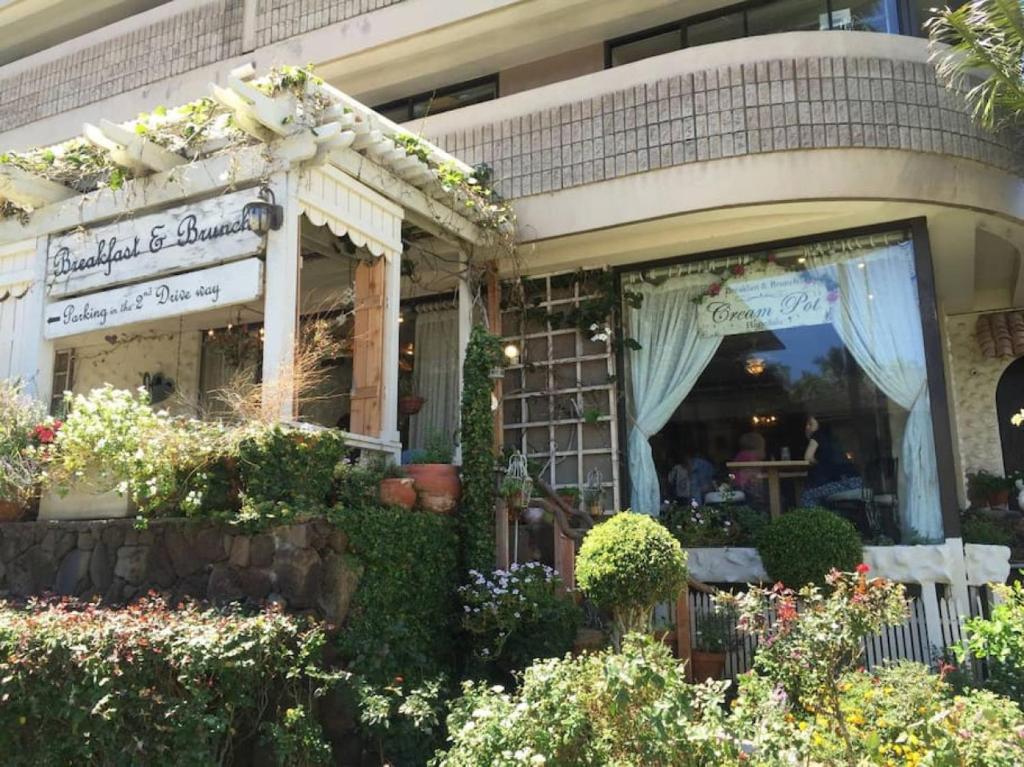The photograph depicts a weather-beaten and old-looking breakfast and brunch place taken during daylight hours, possibly early morning or around noon based on the sunlight. The building features wooden clapboard siding with visible water stains and signs of neglect. At the entrance, a sign indicates "Breakfast and Brunch" and points to parking in the second driveway. The front of the establishment is adorned with a variety of greenery, including bushes, pots, ornamental trees, ivies, and flowers, which mostly obscure the bottom part of the building, leaving only small portions of the stonework visible.

A prominent floor-length glass window on the right side of the image allows a peek inside where two women are seated at a diner's table. Sunlight reflects off both the clapboard and the window, creating a glare that partially obscures a smaller sign inside. Curtains hang behind the window, and inside, other patrons can be seen. A decorative sign reading "Creme Pot" is also visible in or near the large window.